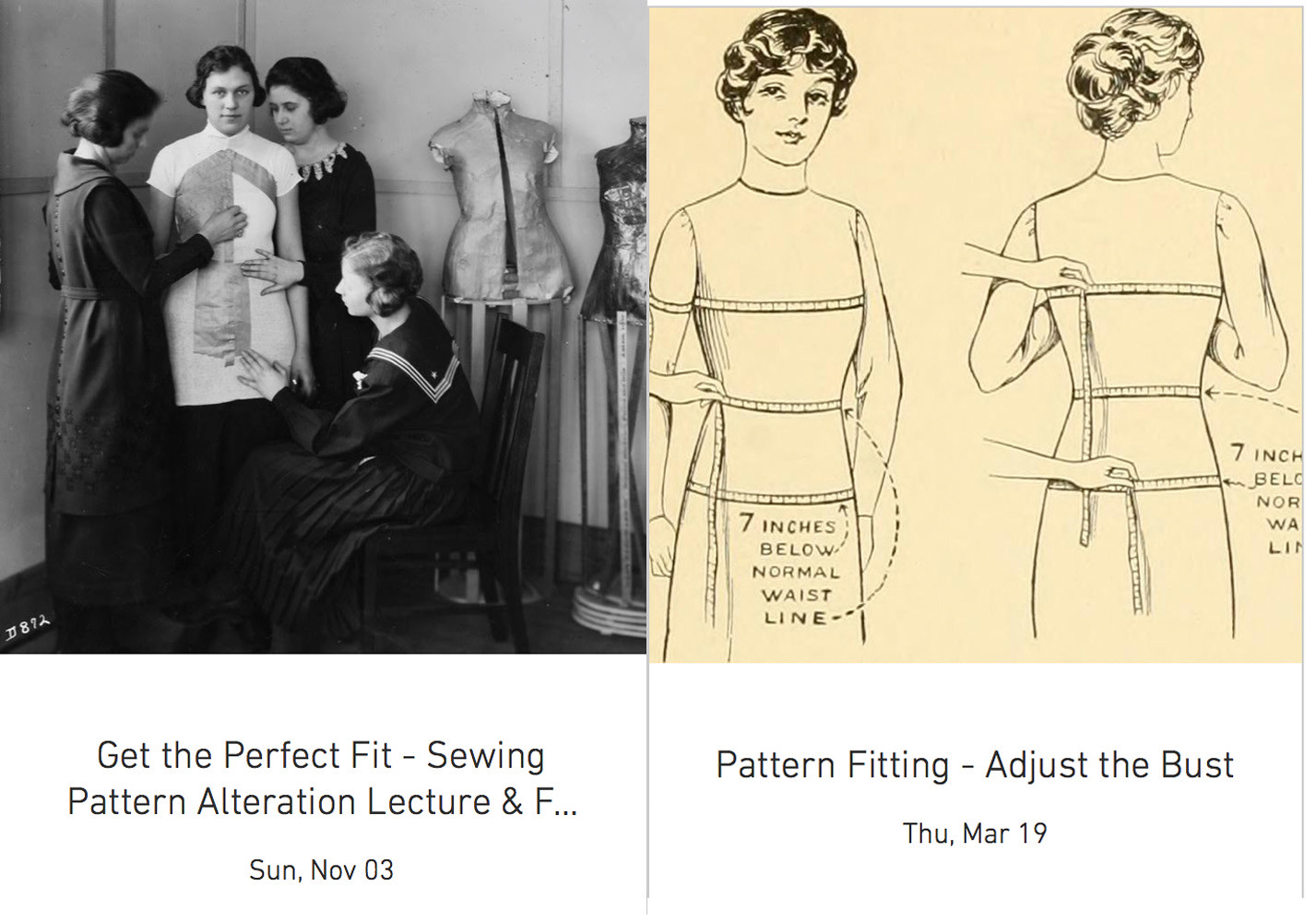This wide rectangular image presents two side-by-side visuals with instructional captions beneath them, set against a white background. The left side features a black and white photograph of a woman standing in a white patterned dress, surrounded by three women in dark, long-sleeved garments. These women appear to be taking measurements and making adjustments to the dress. The caption under this image reads: "Get the Perfect Fit Sewing Pattern Alteration Lecture," with the date partially obscured, indicating "F...Son, November 3rd." The right side showcases a tan background with two drawn images of mannequins, each displaying a woman in a patterned dress. The caption here states: "Pattern Fitting, Adjust the Bust," scheduled for "Thursday, March 19th." In addition, a note points out a specific modification, marking "seven inches below the normal waistline."